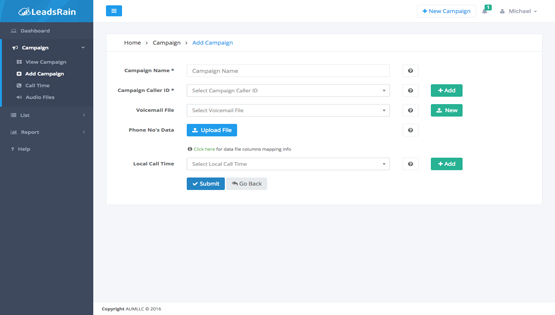This screenshot captures an interface of a web application named "Leads Rain". The app's name is prominently displayed on a blue header bar in white text, also presenting an icon whose details are unclear. Below the header, the left-hand column features a vertical navigation menu on a black background with various options written in white text. The visible options include “Dashboard” at the top followed by “Campaign” in bold, indicating it is currently selected. Next to this, a vertical blue bar emphasizes the selected state. Other options in the menu include “View Campaign”, "Add Campaign", "Call Time", "Audio Files", "List", "Report", and "Help".

The main workspace of the application is dominated by a large gray section containing a substantial white box. At the top, the breadcrumb navigation pathway begins with “Home” followed by "Campaign" and "Add Campaign" highlighted in blue. Beneath this, several input fields are defined with explanatory labels such as “Campaign Name” and “Campaign Color ID”, featuring standard form elements like text boxes, drop-down menus, and help icons denoted by black circles with white question marks.

Fields are effectively delineated, starting with "Campaign Name" accompanied by an input box and a help icon. Below this, "Campaign Color ID" with a drop-down selector and a help icon follows. Another significant section includes "Voicemail Files" with an option to select a file, supported by its drop-down menu and associated help icon, followed by a green box labeled “Add”.

Further down, options include "Phone NO-S Data", a file upload button identified by a blue box with a white profile icon, plus "Local Call Time" with another drop-down menu. Concluding this segment, a “Submit” button in a blue box with a white check mark and a “Go Back” button in a light gray box with a left arrow is showcased.

Above the main workspace is a white header bar spanning the width of the screen. It features a blue hamburger menu on the left and several action icons on the right, including a "New Campaign" button, a notification icon with a green indicator showing the number one, and a profile icon with the name "Michael" alongside a drop-down arrow.

The background outside the main content area remains gray. At the bottom of the image, "Copyright ALUMLLC 2014" is noted in black text, marking the footer of the interface.

This detailed caption underscores the meticulous layout and feature includes of the "Leads Rain" web application screenshot.